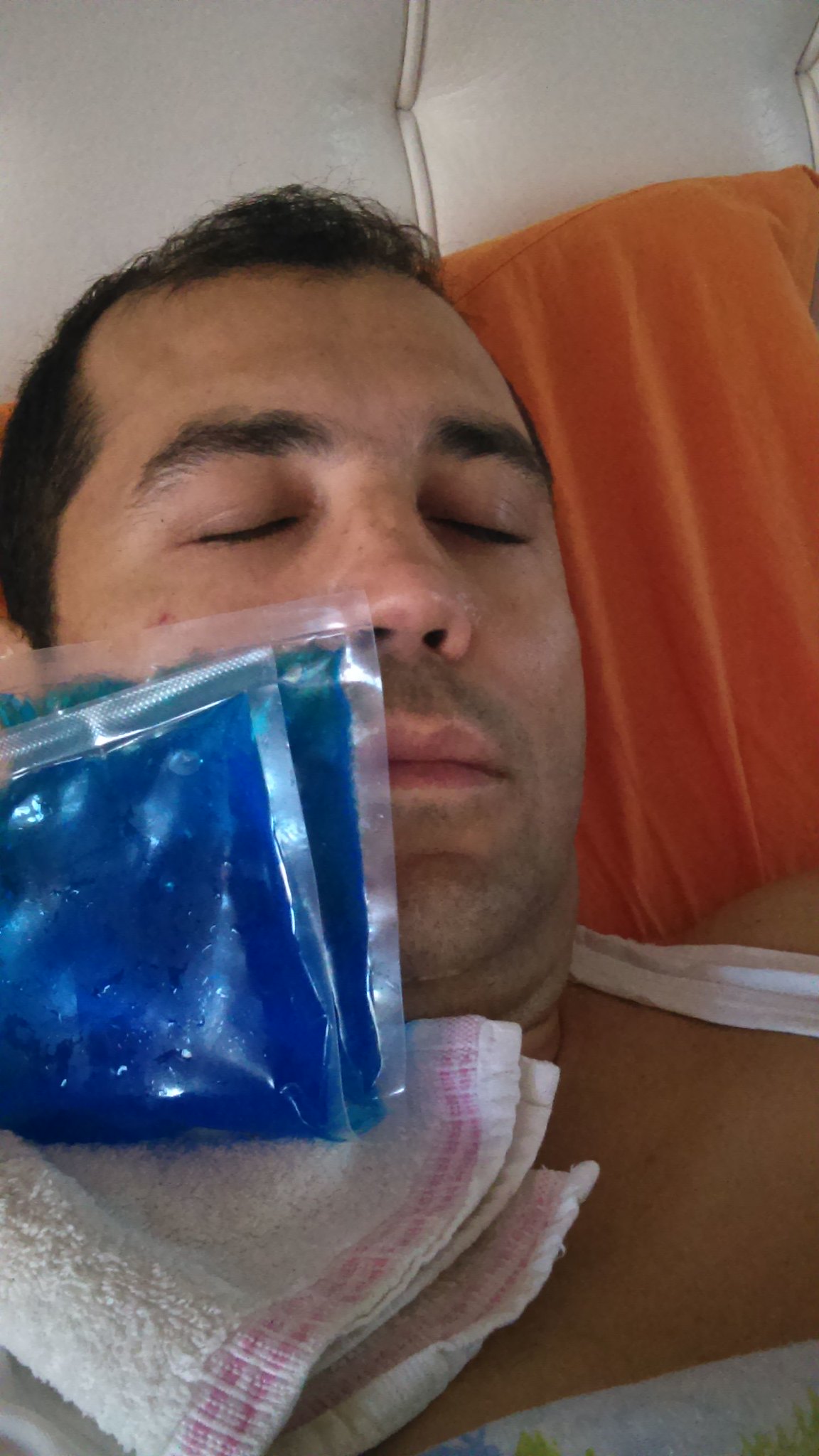In this photograph, a man lies down with his eyes closed on a leather sofa, which features an orange pillow behind him. Appearing to be in his late 30s or early 40s, the man has dark black hair with a subtle receding hairline and a 5 o'clock shadow. He is shirtless, revealing the top part of his chest as well as his neck and shoulders. Resting on his face is a clear plastic blue packet filled with liquid, which is folded in half. The packet is pressed against the lower half of his right cheek, jawline, and sideburn. Beneath the blue packet, there is a folded flannel towel with a rough texture that has a couple of red-pink stripes running along its bottom edge. A strap of bandage-like material extends from the left side of his neck diagonally downwards. In the bottom right corner of the frame, there is a visible piece of material suggesting a blanket or more bandages, indicating he may be recuperating from an injury or medical procedure, most likely involving dental work or a migraine, given the ice pack on his face.